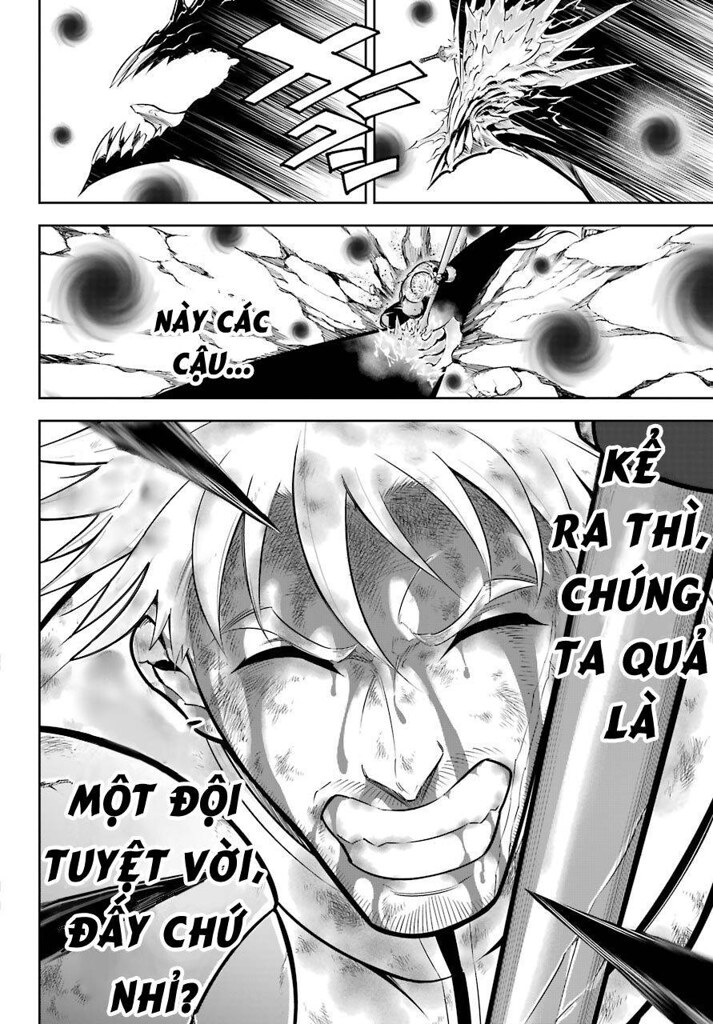The image captures a snippet from a Japanese-style anime comic book drawn in black and white, divided into three sections. The topmost section features chaotic imagery, including wild bangs, swirling lines, and sharp, clawed teeth that suggest the presence of a demon or monstrous figure. Text in a foreign language, possibly Vietnamese, is interspersed within the art. The middle section continues the chaotic theme with dynamic black swirls and more foreign text, likely depicting an intense action scene between the demon and a man. The largest and bottom section zooms in on the man's face, showing him with spiky white hair, eyes closed in a squint, mouth open in a scream, and an expression that conveys pain and exertion, clearly engaged in a fierce struggle.